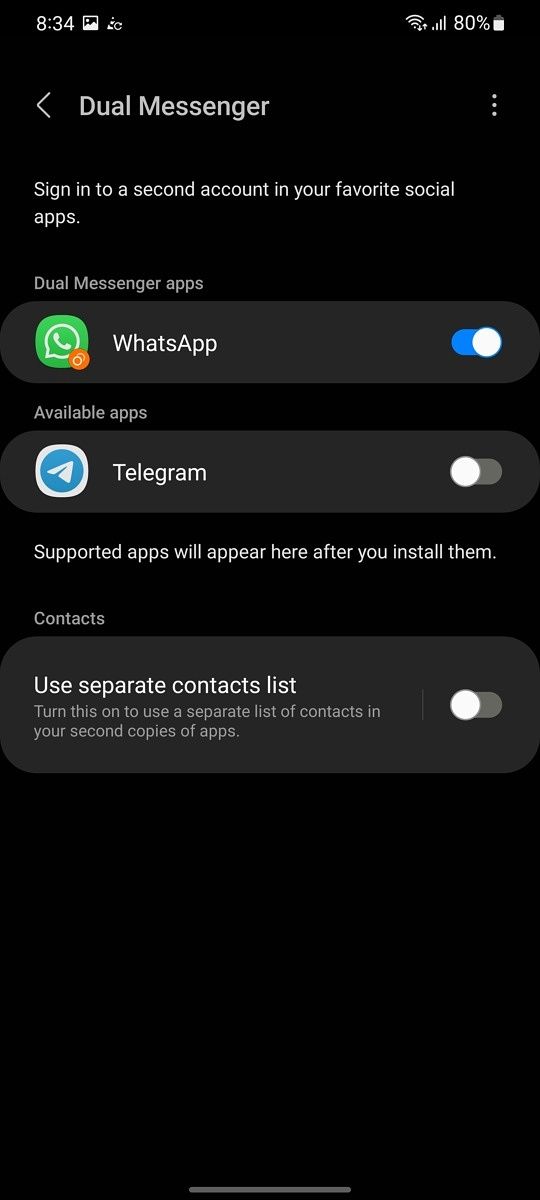Screenshot from an Android phone displaying the WhatsApp app, possibly accessed through the settings menu. The interface shows the "Dual Messenger" feature, allowing users to sign in to a second account on supported social apps. The title of the page reads "Dual Messenger," with a subtext stating, "Sign in to a second account in your favorite social apps."

Underneath, there are toggles for WhatsApp and Telegram. The toggle next to WhatsApp is switched on, indicating a second account is active. The toggle for Telegram is switched off. Additionally, the screen includes a note that supported apps will appear in this list after installation, but Telegram remains disabled for dual usage.

Below these settings, there's an option to activate a "Separate contacts list," which allows the user to maintain distinct contacts for their second app accounts. This option is currently not enabled.

The screenshot was taken at 8:34, with the battery level at 80%, and the WiFi connection appears to be functioning well.